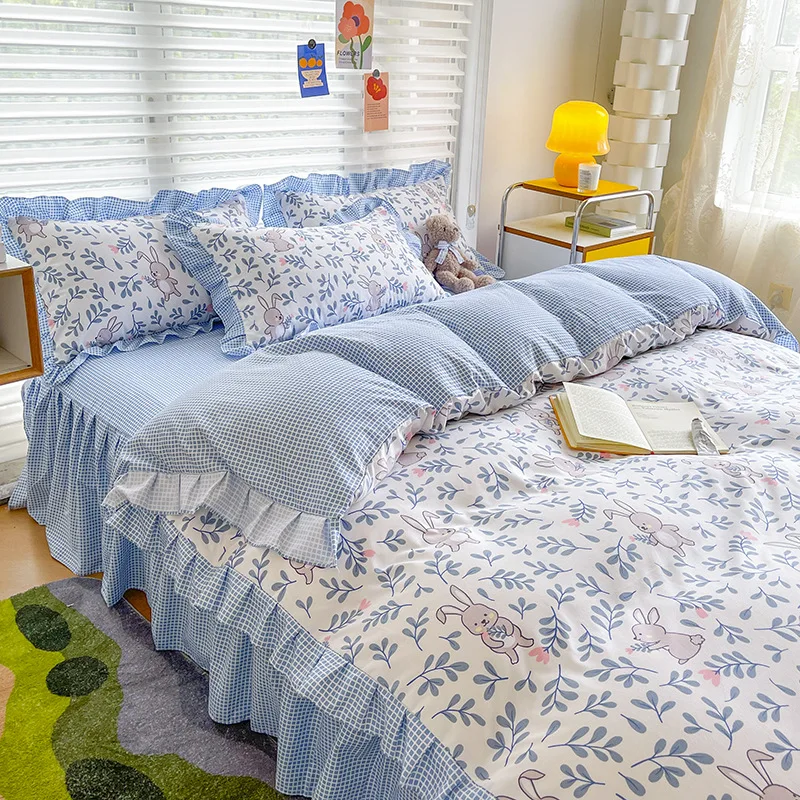This photo depicts a charming and whimsical children's bedroom centered around a full-sized bed draped with a blue and white checkered flannel comforter adorned with patterns of tan and brown bunnies and green leaves. The bed is further accented by three matching flannel pillows featuring the same delightful bunny and leaf design. A cuddly teddy bear with a bow tie sits prominently on the left side of the bed next to an open book, suggesting a space ready for bedtime stories. To the left of the bed, a wooden nightstand holds an orange lamp and a candle, adding a warm hue to the room. The bottom left corner reveals a green and blue rug, complementing the overall color scheme. The back wall showcases a large picture window flanked by blinds, with three small paintings—two of flowers and one of a pot—hanging neatly against the shades. The natural light streaming through the windows enhances the room's serene and inviting atmosphere.